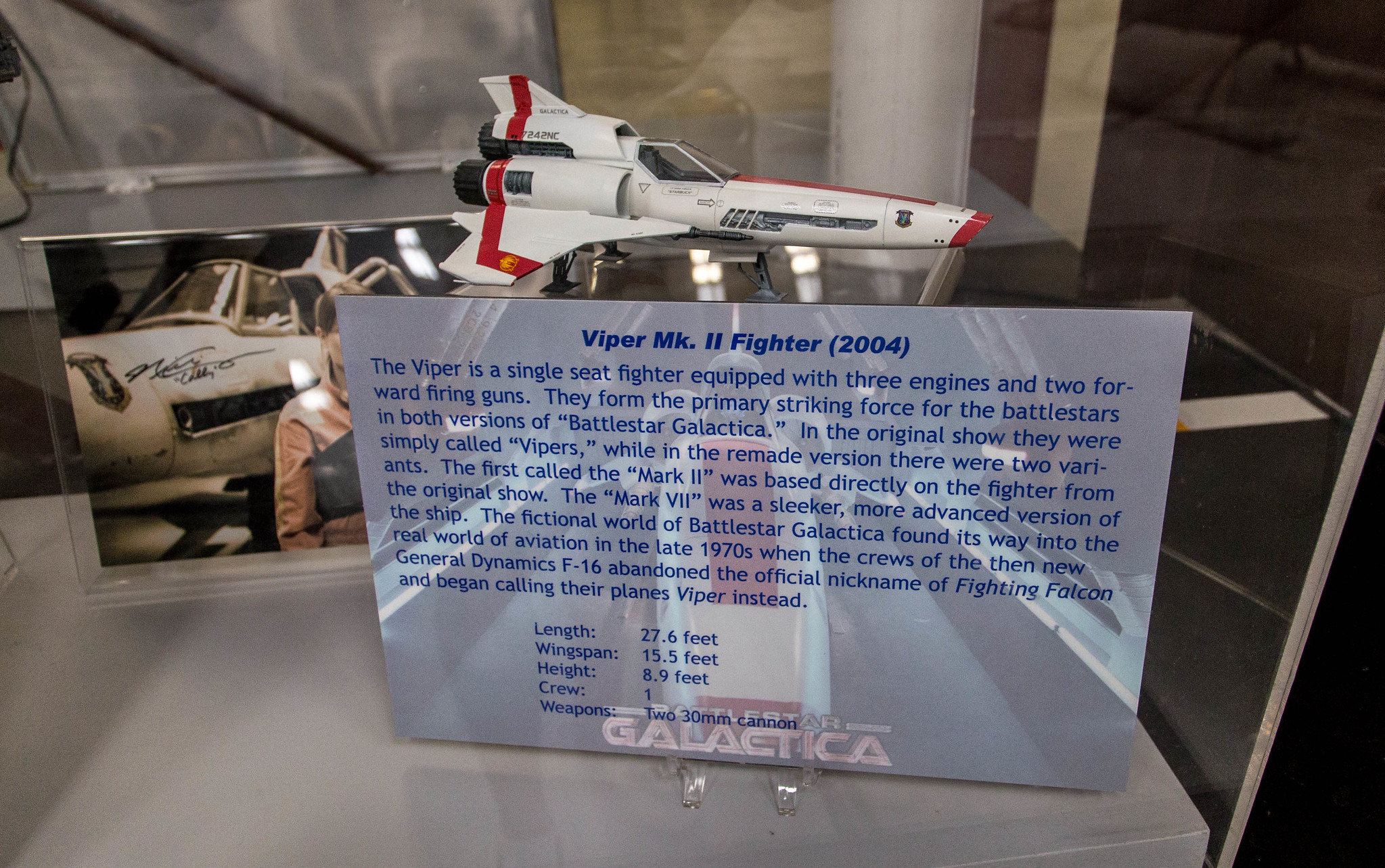The image depicts a detailed display within a museum setting, focused on the Viper Mk II Fighter from the television series Battlestar Galactica. Encased in plexiglass, the display sits on a clean, gray table. The exhibit includes a meticulously crafted model of the Viper Mk II, which is predominantly white with red accents, featuring a red stripe on the back and a red front end, exuding a futuristic starship aesthetic. Adjacent to the model, there's a photograph with a brown hue illustrating a pilot posing with a prop ship, emphasizing the display's connection to the show. 

Behind the model, a blue informational plaque provides comprehensive details about the Viper Mk II. The text, written in blue, states that the Viper is a single-seat fighter armed with two forward-firing guns and equipped with three engines, functioning as the primary strike force for the Battlestars in both iterations of Battlestar Galactica. The plaque also references that the original Vipers inspired the Mk II version, while later shows introduced a more advanced Mk VII variant. Additionally, it mentions the influence of Battlestar Galactica on real-world aviation, noting that the pilots of the General Dynamics F-16 adopted the nickname "Viper" for their aircraft. The placard includes technical specifications: length of 27.6 feet, wingspan of 15.5 feet, height of 8.9 feet, crew capacity of one, and armament consisting of two 30-millimeter cannons. The exhibit is set against a dark, black far-side wall with a metallic element visible in the background, enhancing the overall ambiance of the display.